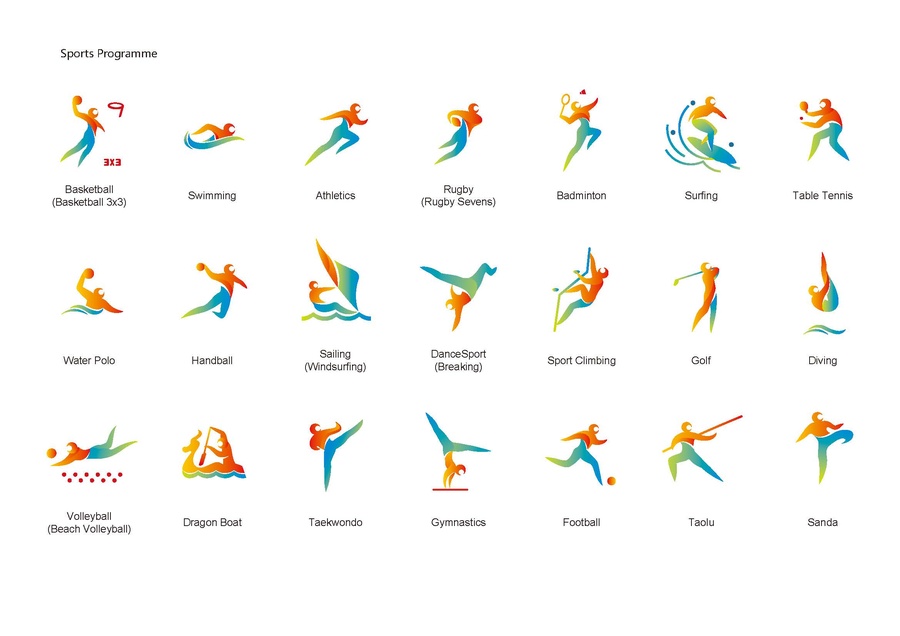The image is a detailed chart entitled "Sports Program" situated at the top left. It features orange and blue human-shaped icons illustrating various sports activities, arranged in rows. The first icon depicts a basketball player executing a slam dunk into a hoop, labeled as "Basketball 3x3." Adjacent to it, there's a swimmer portrayed within a swish of water, labeled "Swimming." Following that is a runner labeled "Athletics" and a rugby player carrying a brown egg-shaped ball, labeled as "Rugby Sevens." Additional icons include figures performing badminton, surfing, table tennis, water polo, handball, and sailing (with windsurfing in parentheses). Furthermore, icons for dance sport (breaking), sport climbing, golf, diving, volleyball, dragon boat racing, taekwondo, gymnastics, football, taolu, and sanda are also depicted, each figure uniquely posed to represent its respective sport.